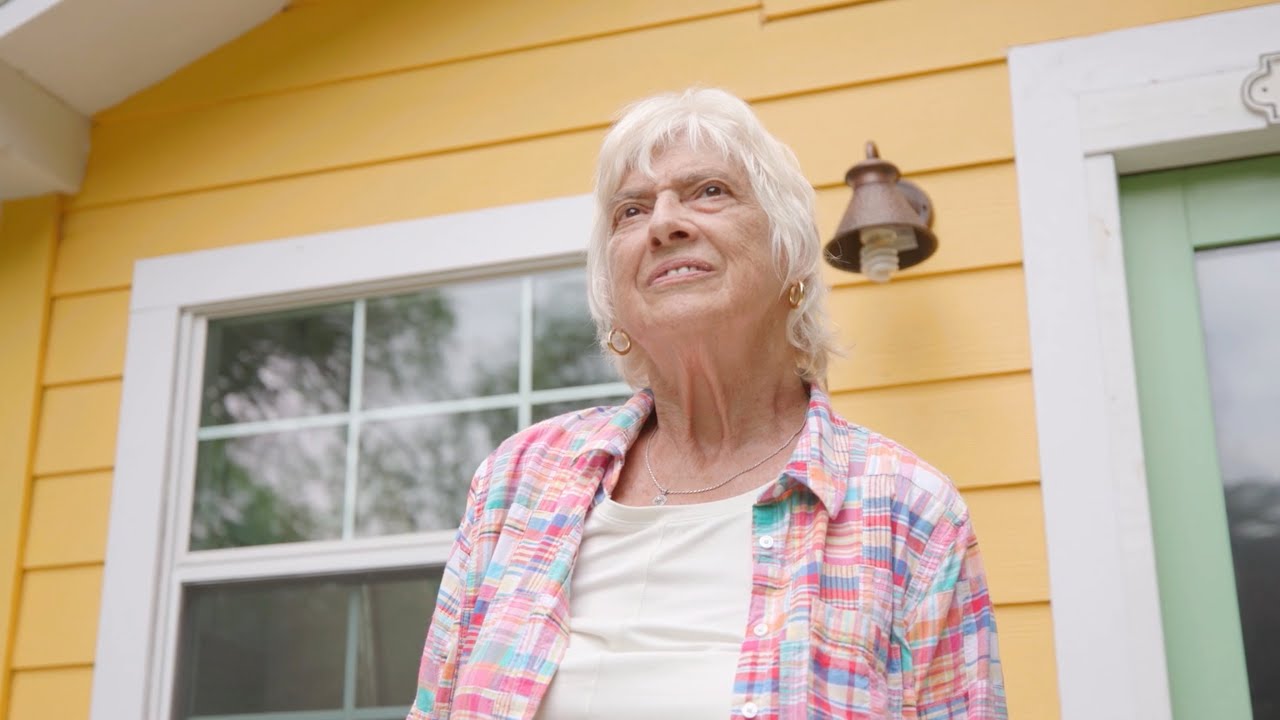This photograph captures an older woman standing on her porch, taken from a lower angle which accentuates her presence against the backdrop of her yellow-painted house. She has white hair and is adorned with small gold hoop earrings and a silver necklace. The woman is warmly smiling and dressed in a multicolored checkered shirt over a white T-shirt with a hint of yellow. The house features white window frames and a white door frame, with the door itself painted a light green. A bronze light fixture is mounted between the window and the door, adding a subtle glow to the scene, which emphasizes the welcoming and serene atmosphere. The woman, standing confidently as the focal point of the image, brings a sense of homeliness and warmth to the photograph.